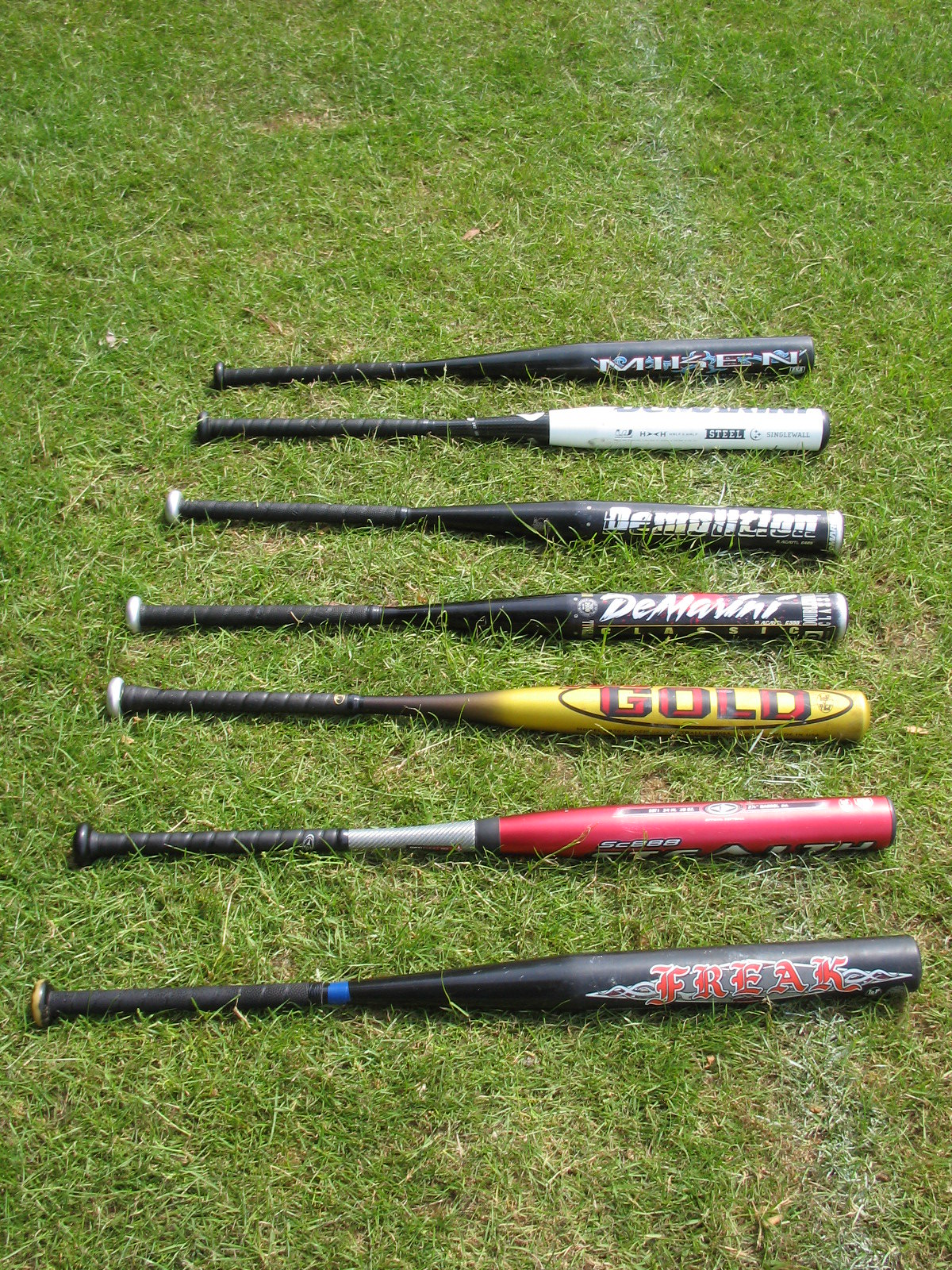In the foreground of the image, which captures a large, dark green grass field under the mid-afternoon sun, seven baseball bats are meticulously laid out in a vertical line, spanning from the top to the bottom of the frame. The first bat is entirely black with white lettering that reads "Minkin." The second bat features a white handle with a predominantly black body. The third bat is black with bold white text that says "Demolition." The fourth bat continues this theme and also has a black body with white lettering that spells out "Demarini." The fifth bat stands out with its intricate design—it has black strap lines on the handle, a gold top, a black line around the middle, and large red letters that read "GOLD." The sixth bat has a complex color scheme with a black-lined bottom, a grey middle, and a reddish top. Finally, the seventh bat, positioned at the bottom of the lineup, combines dark grey straps and a light blue section near the handle, transitioning into a black bat with red letters spelling "Freak." These bats, each unique in design and color, are carefully arrayed on the grass, creating a striking visual contrast against the verdant background.